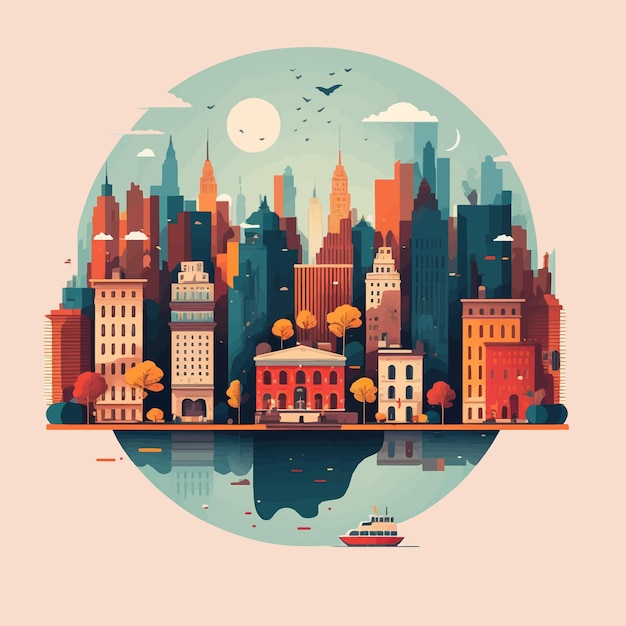This detailed watercolor painting depicts a vibrant cityscape, likely representing New York City, with emphasis on a skyline reminiscent of Manhattan. The scene features a variety of skyscrapers and smaller buildings, all realistically rendered with a bright array of colors including oranges, yellows, and multiple shades of blue. The city section appears encased as though in a snow globe, set against a cream-colored background. A large body of water lies in the foreground, reflecting some of the high-rises and a small ferry boat, alongside a few other objects. The painting also captures golden and red trees, suggesting a fall setting. Above the cityscape, the artwork includes birds, low-lying cumulus clouds, and both a sun and a crescent moon, adding to the overall whimsical yet realistic feel of the piece. The presence of the Metropolitan Museum of Art and its reflection are subtly integrated, reinforcing the New York City essence of the painting.